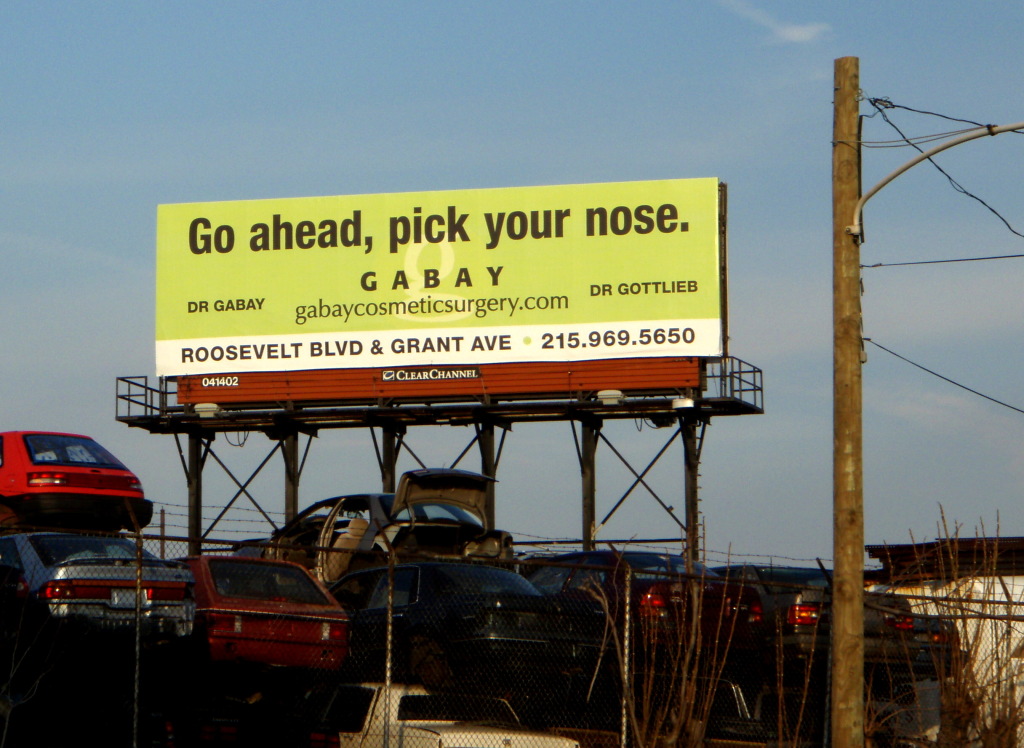Under a brooding, cloudy sky with a hint of blue peeking through at the top, a weathered wooden telephone pole rises from the ground, festooned with numerous wires. The scene is dominated by a large, eye-catching billboard. The billboard features a yellow rectangle at the top and a white rectangle at the bottom, both adorned with bold black text. The top section of the text humorously reads, "Go ahead, pick your nose," followed by the endorsement "Gabby," spelled out as G-A-B-B-Y. The bottom left corner identifies "Dr. Gabby," while the bottom right corner introduces "Dr. Gottlieb." Above these names, the URL "G-A-B-Y cosmetic surgery dot com" is prominently displayed, and below the main text, the location is given as "Roosevelt Boulevard and Grand Avenue," with a contact number, "215.969.5650." The Clear Channel brand is marked at the very bottom of the billboard.

The setting of this scene appears to be a junkyard, where a chaotic assortment of cars is stacked atop one another. One car has its trunk open, and another is missing a door, adding to the atmosphere of disarray. A fence topped with barbed wire encloses the junkyard, emphasizing the gritty, industrial nature of the environment.